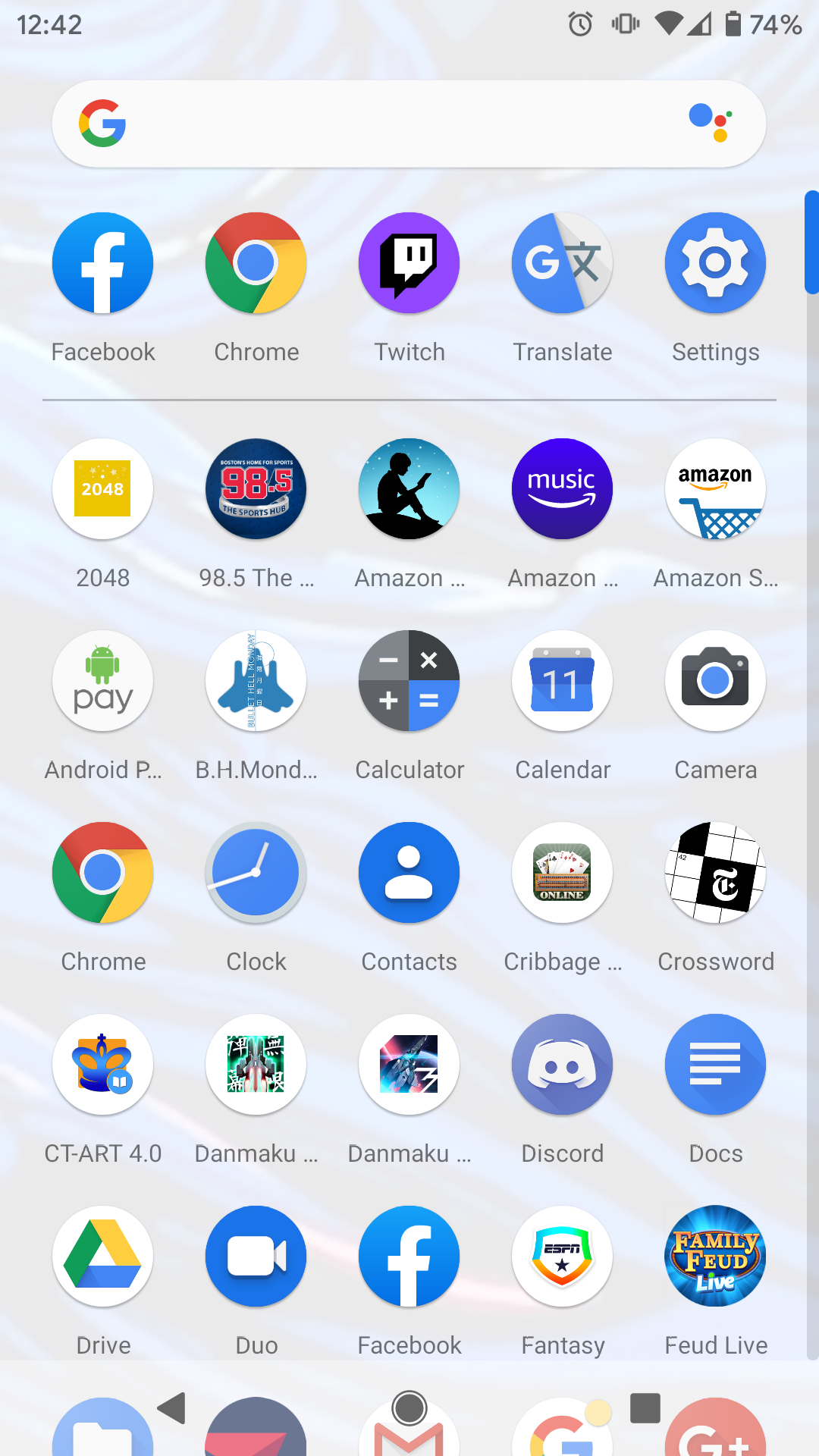The image depicts an Android home screen filled with a myriad of selectable app icons. The background features a faded paisley pattern in shades of blue, black, and white, subtly enhancing the visual overall. At the very top, the status bar provides key information: the time is displayed as '12:42' on the right, and moving leftwards from the center, there are icons for a clock, a vibrate mode indicator, a fully-colored WiFi signal, and a half-filled phone network signal represented by a right triangle. The battery icon shows it's three-quarters full at 74%.

Beneath the status bar lies the Google search widget, featuring the Google 'G' logo, an empty search bar, a blue ball, and a profile picture icon to the left. Directly below this are shortcuts to apps like Facebook, Chrome, Twitch, Google Translate, and Settings.

Further down, six rows of app icons are organized neatly:

1. **Row 1**: 2048 game, 98.5 radio station, Amazon Kindle, Amazon Music, Amazon Shopping, Android Pay.
2. **Row 2**: BH Monday, Calculator, Calendar, Camera, Chrome, Clock.
3. **Row 3**: Contacts, Cribbage, New York Times Crossword, CT-ART, two different Domicode apps.
4. **Row 4**: Discord, Google Docs, Google Drive, Duo, Facebook, Fantasy.
5. **Row 5**: Family Feud Live.
6. **Row 6**: Partially visible icons, including the tops of documents, the Delta symbol, the Gmail icon, the Google logo, and the Google+ symbol.

Each app icon is clear and distinct, indicative of the diverse range of functionalities and entertainment available at the user's fingertips.